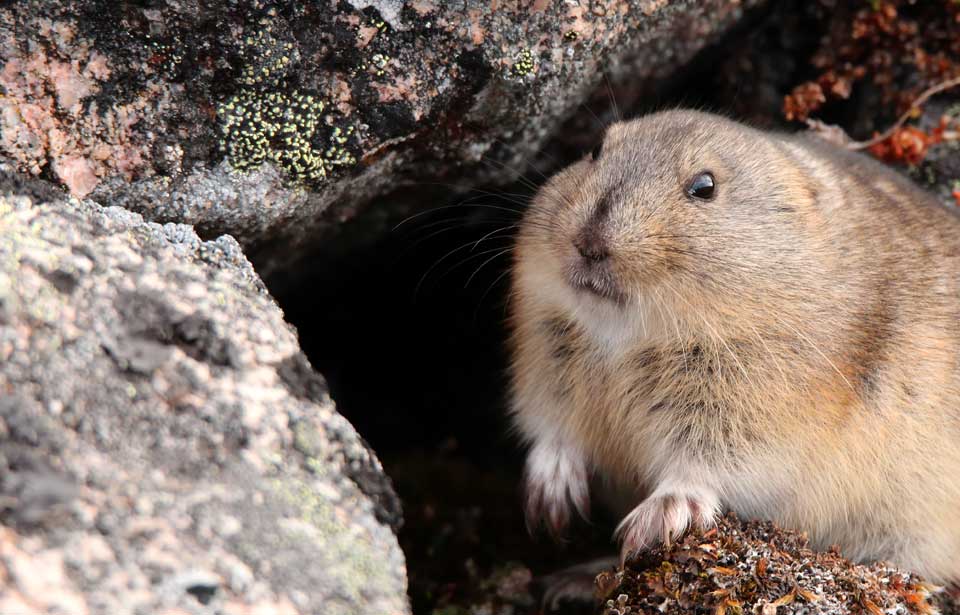In the photograph, a large, stout rodent—likely a marmot or a groundhog—peeks out from between a formation of large, stacked boulders. The animal has a rotund body with stubby legs that are barely visible beneath its ample belly. Its fur is predominantly brownish-gray with a mix of white, varying shades of brown, and hints of black, particularly upon closer inspection. The fur is slightly longer on its underside, and there is a distinct white collar under its head and across its belly. The creature has tiny ears positioned towards the back of its head, black beady eyes, and a stout nose that almost blends into its face, complemented by whiskers and a mouth resembling a black line. The boulders around it are adorned with patches of green moss, red-tinted dry leaves, and whitish-red lichen, giving the impression of an outdoor scene rich in texture. The space between the rocks is shadowy and dark, suggesting a potential burrow or hideout for the animal. The marmot appears to be resting one paw on a rock, surveying its surroundings from its natural alcove.